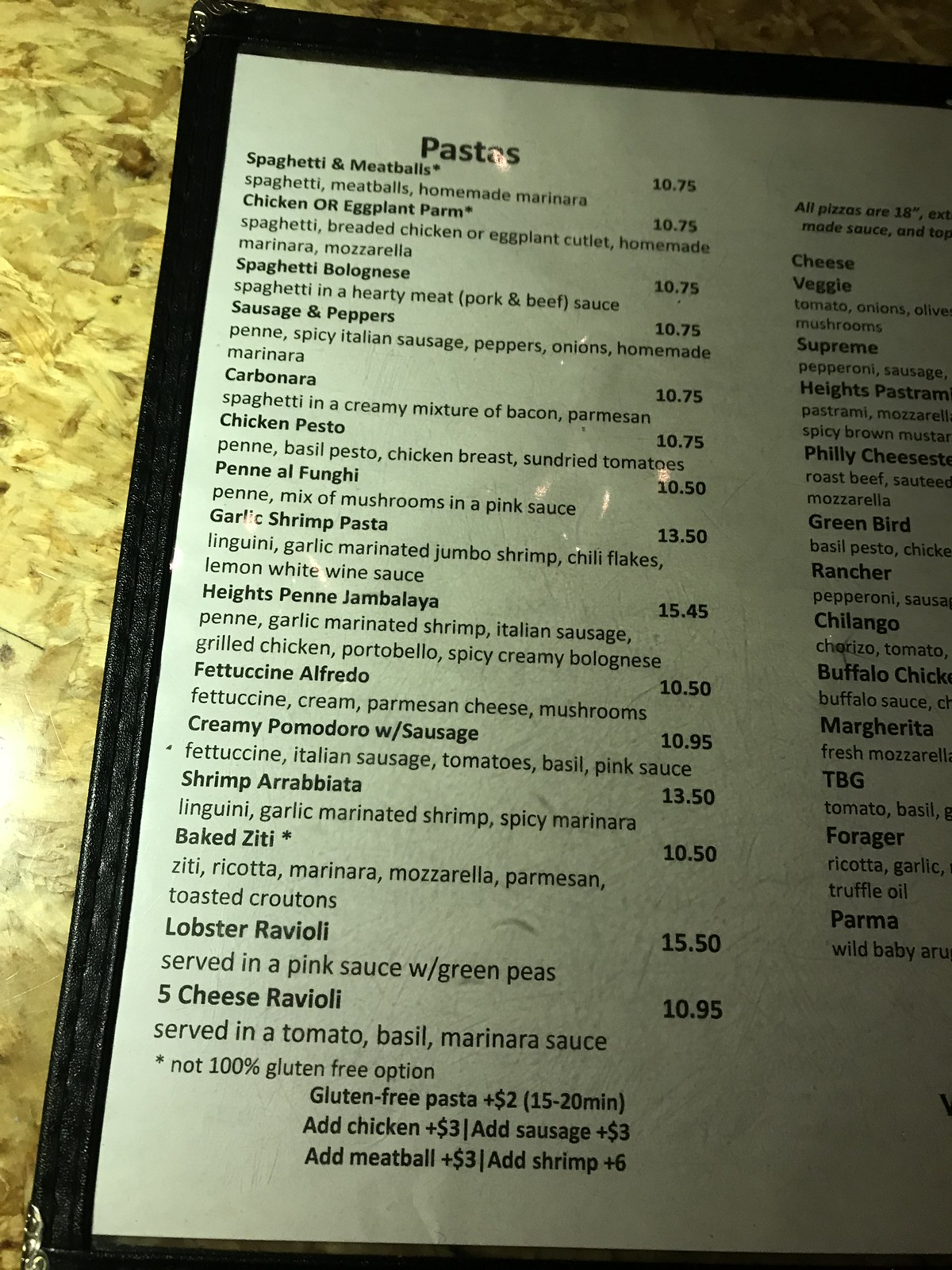This image showcases a section of a menu page from what appears to be an Italian restaurant. The menu page is partially cropped on the right side, revealing only one column of food offerings. The list features several pasta dishes, each written in black letters with prices indicated next to them on a clean, white background. The paper menu is encased in a transparent plastic cover, with a black frame bordering the visible long left side and shorter top side.

The clearly readable pasta offerings start at the top with "Spaghetti and Meatballs" and end at the bottom with "Five Cheese Ravioli." Other prominent dishes in the column include "Lobster Ravioli," "Baked Ziti," "Fettuccine Alfredo," "Carbonara," "Chicken Pesto," and "Spaghetti Bolognese." The prices for these dishes range from $10.75 for the Spaghetti and Meatballs to a maximum of $15.50 for the Lobster Ravioli.

Although partially obscured, a second column to the right lists various cheese-based dishes, with names like "Veggie Cheese," "Rancher," "Buffalo Chicken," and "TBG." The menu is placed on a table, which is only partially visible within the frame of the image.

Through the selection of traditional Italian dishes and their corresponding prices, the menu suggests that the restaurant offers a range of affordable, classic Italian cuisine.